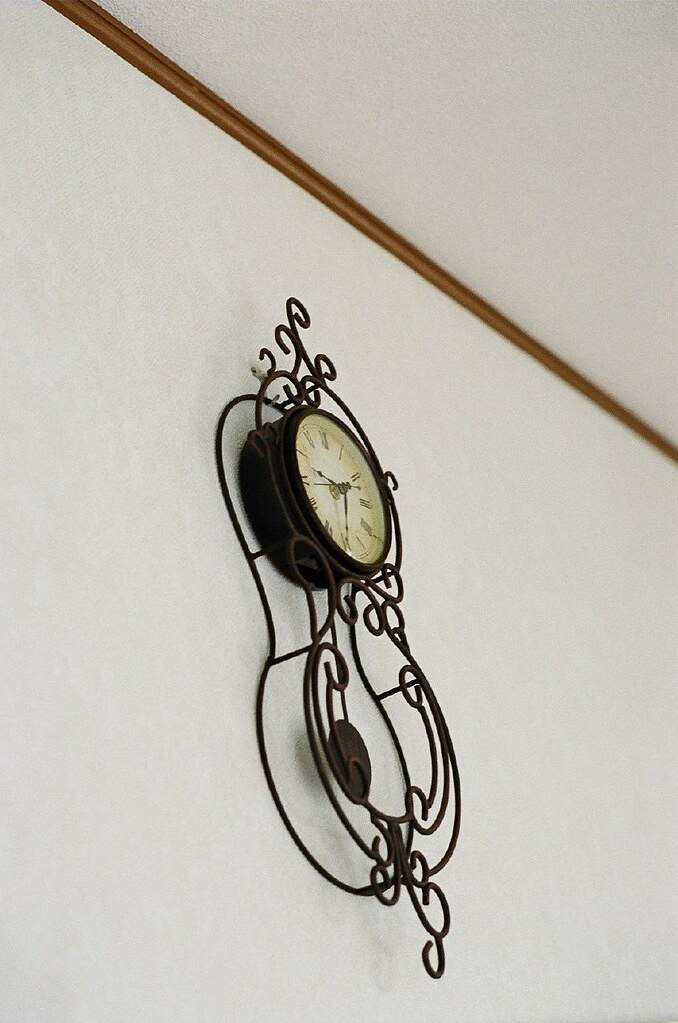The image depicts an ornate, antique-style metal clock hanging on a rough-surfaced white wall, with a matching white ceiling visible in the upper right corner. Separating the wall and ceiling is a dark brown wooden trim. The clock, shaped like a cello or violin with intricate swirl patterns and decorative loops on the top and bottom, features a rustic brown metal frame. The center of this intricate frame houses a black-cased clock with an off-white face marked by black Roman numerals from 1 to 12. The clock also has black hands for the seconds, minutes, and hours.